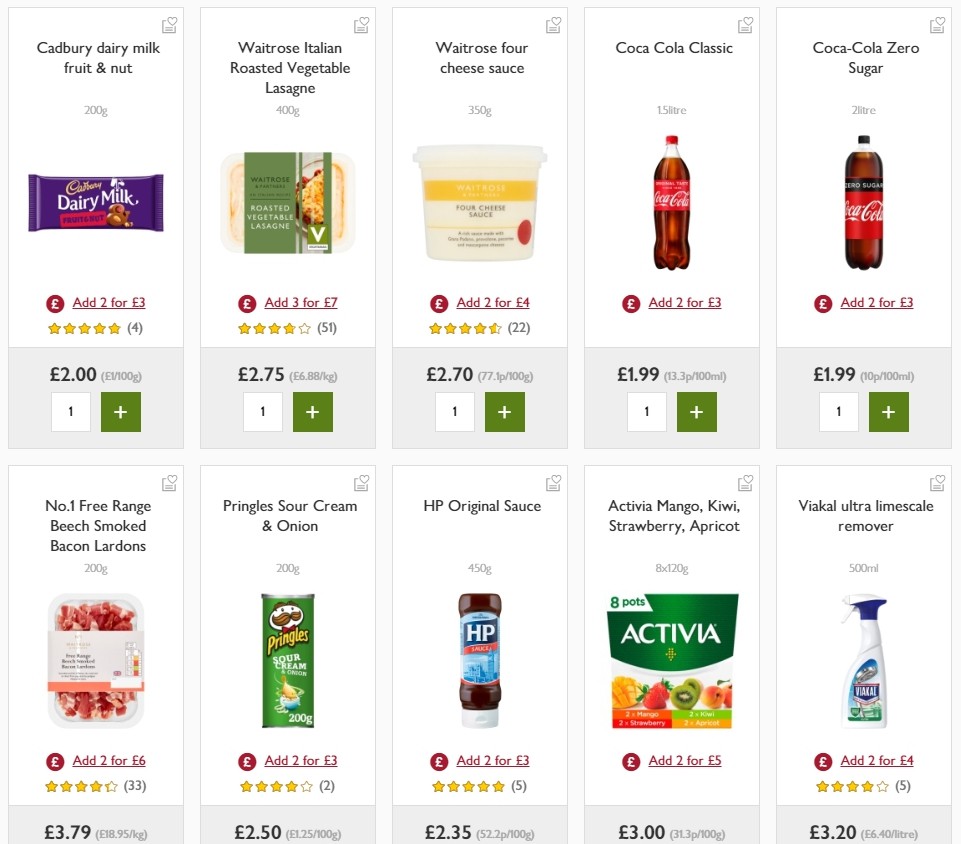Screenshot of an online grocery retail webpage displaying two rows of product listings, with five items per row. Each product is presented in a vertical rectangular block containing the product name, an image, a rating, the price per unit, and options to adjust quantity and add to the cart.

In the upper left block, there is a 22-gram Cadbury Dark Milk Fruit and Nut candy bar. The product boasts a five-star rating from four reviews and is priced at £2.00 per unit. To its right, the next item is Witch Roast Italian Roasted Vegetable Lasagna, which weighs 400 grams. The product image is displayed, accompanied by a promotion to add three for £7.00. This lasagna has earned a four-star rating from 51 reviews and is individually priced at £2.75.

Continuing along the upper row, the assortment includes a Coca-Cola product, a cheese item, suggesting a diverse selection available.

The bottom row mirrors the layout of the upper row. It starts with a pack of bacon to the left, followed by a variety of chips. Further to the right, a soda, a product featuring strawberry and kiwi flavors, and finally, a limescale remover.

Each product block includes details such as the name, image, rating, price, and quantity adjustment options, typical for online grocery shopping platforms.